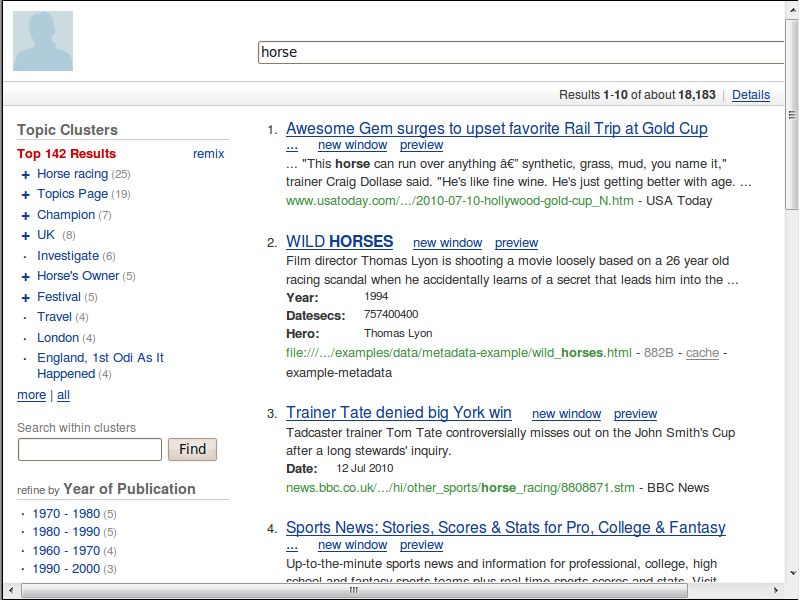The image features a visually organized interface on a white background. Along the left and top edges, there is a green border, while the right side features a blue vertical slider with up and down arrows and three horizontal lines on it. At the bottom of the image, there is a similar blue horizontal slider with left and right arrows and three horizontal lines in the middle.

At the top of the interface, a blue square depicts the outline of a person, next to which a search box contains the word "horse." Following this, a blue box displays "results 1 through 10 of about 18,183" with a line and the word "details," which is underlined in blue.

On the left side, there is a section labeled "Topic Clusters" with "top 142 results" in red text and "remix" in blue. The topics listed include "horse racing," "topics page," "champion," "UK," "investigate," "horses owner," "festival," "travel," "London," "England," "first OD as it happened," "more," and "all." Below these topics, there is another search box alongside a "find" button and options to refine the search by "year of publication" ranging between 1970 and 2000.

On the right side, the results are enumerated:
1. "Awesome Gym Surges to Upset Favorite Rail Trip at Gold Cup"
2. "Wild Horses" with "new window" and "preview" underlined
3. "Trainer Tate Denied Big York Win" with "new window" and "preview" underlined
4. "Sports News: Stories, Scores, and Stats for Pro, College, and Fantasy" with "new window" and "preview" underlined.